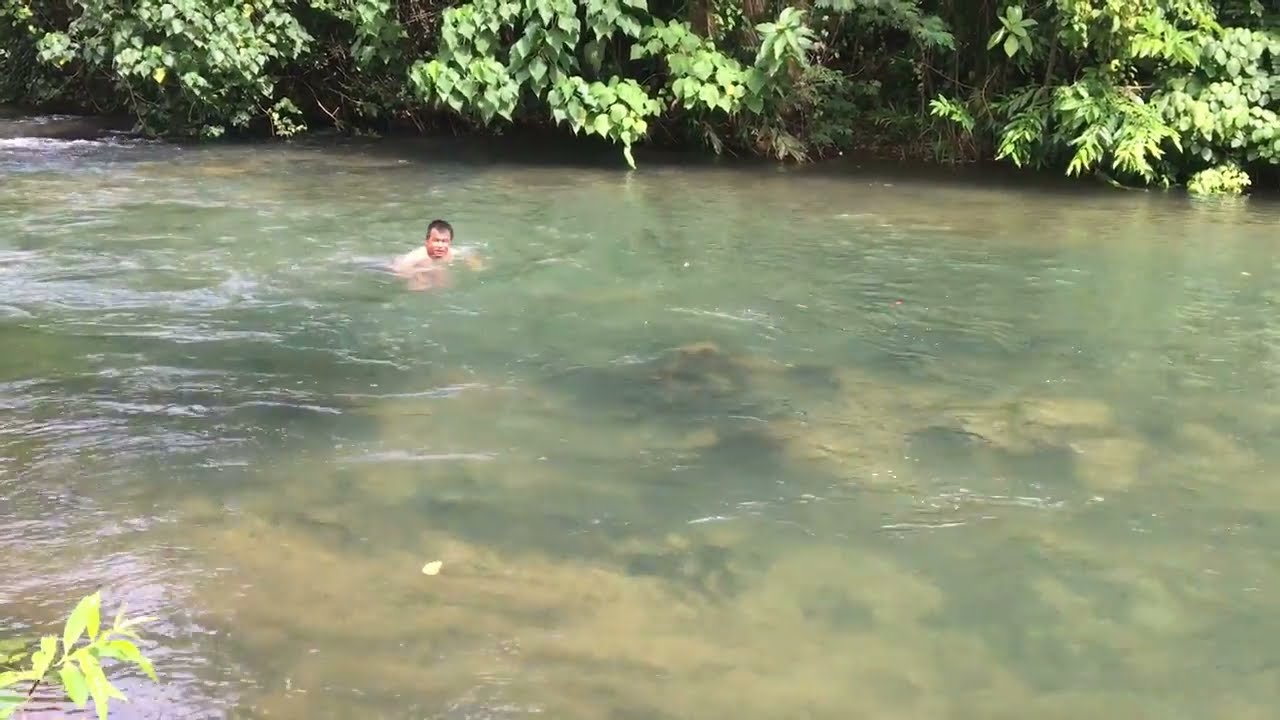A young Asian man, appearing to be about 30 years old, is captured swimming in a clear, greenish lake or river under the warmth of a sunny day. The water, slightly mottled with brown patches and white wave reflections, suggests cleanliness and a transparency that almost reveals the bottom. The man, stocky with short black hair, is in the midst of a swimming motion—potentially a backstroke or transitioning to a forward swim—with no one else in sight. Surrounding him, the banks of the water body are lush with green plants, tree leaves, and possibly branches dipping into the water. The scene, reminiscent of locations like Thailand or the Philippines, encapsulates a serene and solitary moment of leisure in nature.